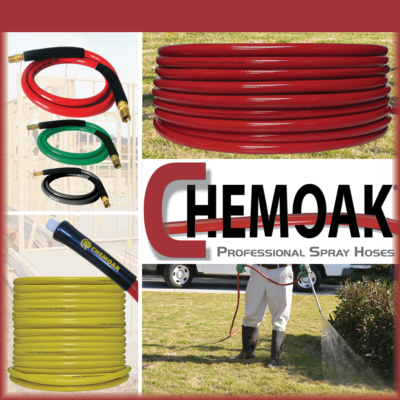The square advertisement prominently features the "Chem Oak Professional Spray Hoses" branding in the center, with a large red "C" stylized like a bent hose and the rest of the lettering in black, threaded with a red hose. Surrounding this central logo are four distinct images: 

- At the top left, three hoses in descending sizes and colors (red, green, and black) are stacked against a light backdrop.
- Beneath this, on the bottom left, is a yellow hose neatly coiled on a reel, with a detailed close-up of the hose end above it.
- The top right image displays a red hose coiled neatly on a bed of grass, showcasing its vibrant color and durable material.
- Below this, the bottom right image depicts a man in white pants and black boots using a red hose to spray a lawn, with a white truck and a nearby bush in the background.

The red border that frames the image is slightly thicker at the top, adding emphasis to the vibrant and dynamic presentation of the spray hoses, which are available in four colors and showcased in practical and appealing settings.